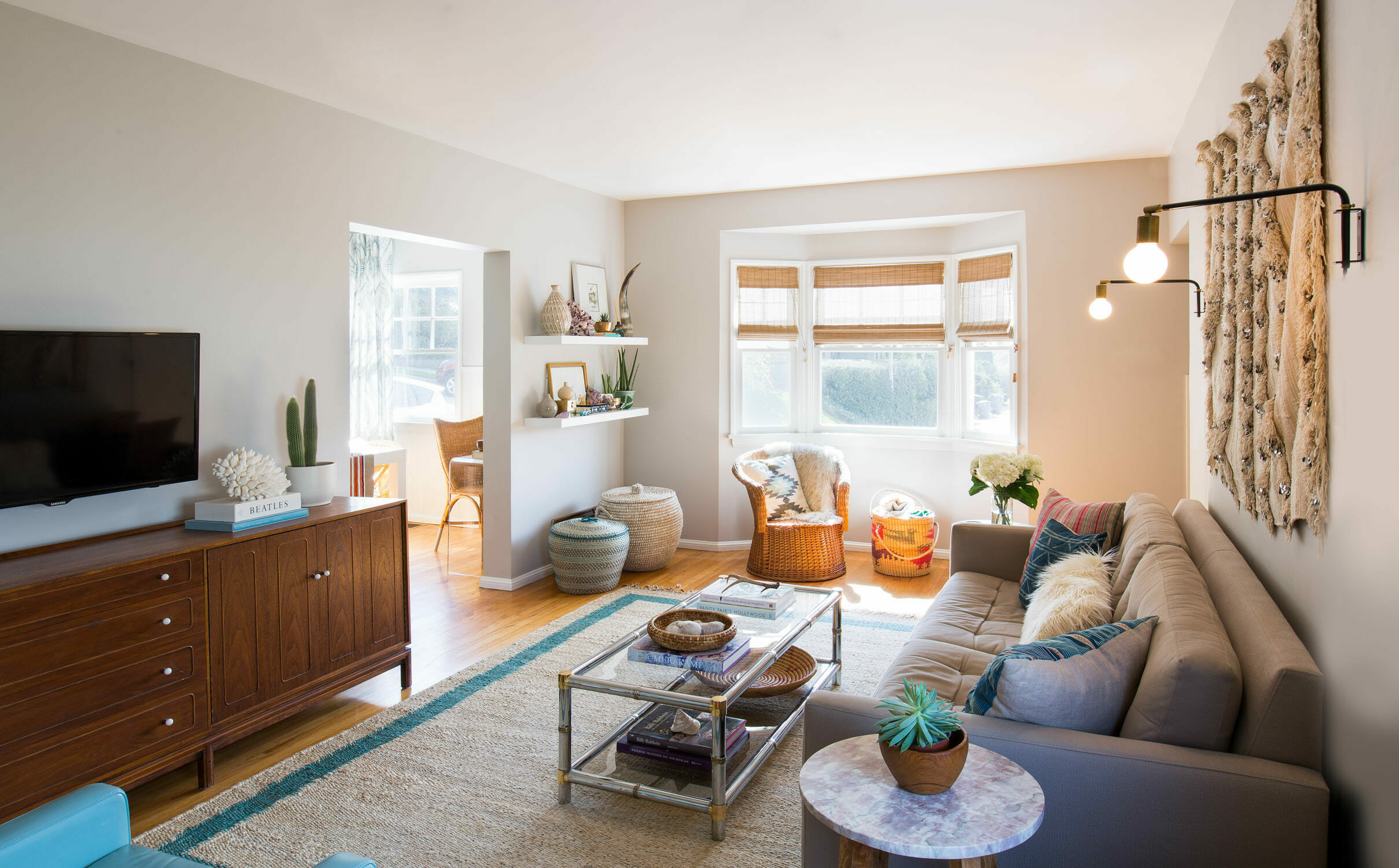This modern, contemporary living room is bathed in natural light streaming through a bay window and an arched entryway, revealing glimpses of a neighboring house and lush hedges. The room features a gray, non-poofy couch positioned against a wall adorned with a hanging tapestry and bracket-mounted lights that can swivel horizontally. The accent wall by the window is a contrasting beige, while the rest of the walls are painted light gray, providing a sophisticated backdrop to the space. 

A long wooden console with four drawers and doorknobs beneath a mounted flat-screen TV anchors the room. Decoratively, it holds a white book titled "Beetles" alongside ornamental flowers, a cactus in a white pot, and a large piece of white coral. Flanking the bay window are two wall shelves filled with knickknacks, plants, pots, and framed art, while wicker or ceramic baskets sit beneath.

In front of the couch, a modern coffee table with a glass surface supported by faux bamboo railings in silver and gold metal serves as a centerpiece. A large cream-colored rug with a green trim border underpins the seating area, complementing the decor. Opposite the couch, there's a side table with a green plant on it. A rattan chair adorned with Southwestern-style throw pillows and a side table topped with marble add to the room’s eclectic charm. The wooden floor ties everything together, creating a warm, cohesive look.